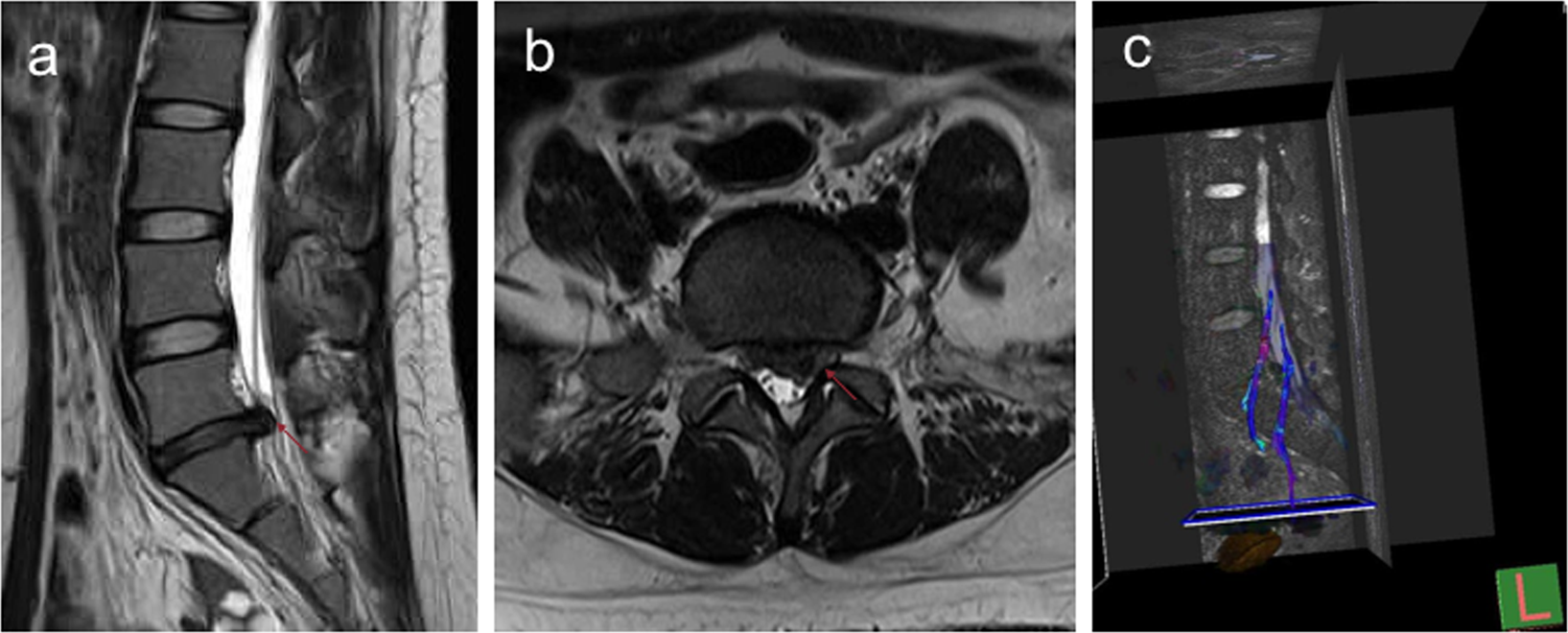The image consists of three distinct parts, labeled A, B, and C in the upper left of each segment. They resemble medical imagery, possibly x-rays. The photo is primarily in black and white except for part C which contains some color. In part A on the left, numerous rectangular segments create a pattern suggestive of spinal discs aligned vertically. Part B, centered, features a round, possibly cross-sectional view that could depict a single spinal bone or a pelvis. Part C on the right incorporates some blue lines that resemble veins or anatomical markers, and includes a green box with a pink 'L', adding to its diagnostic nature.